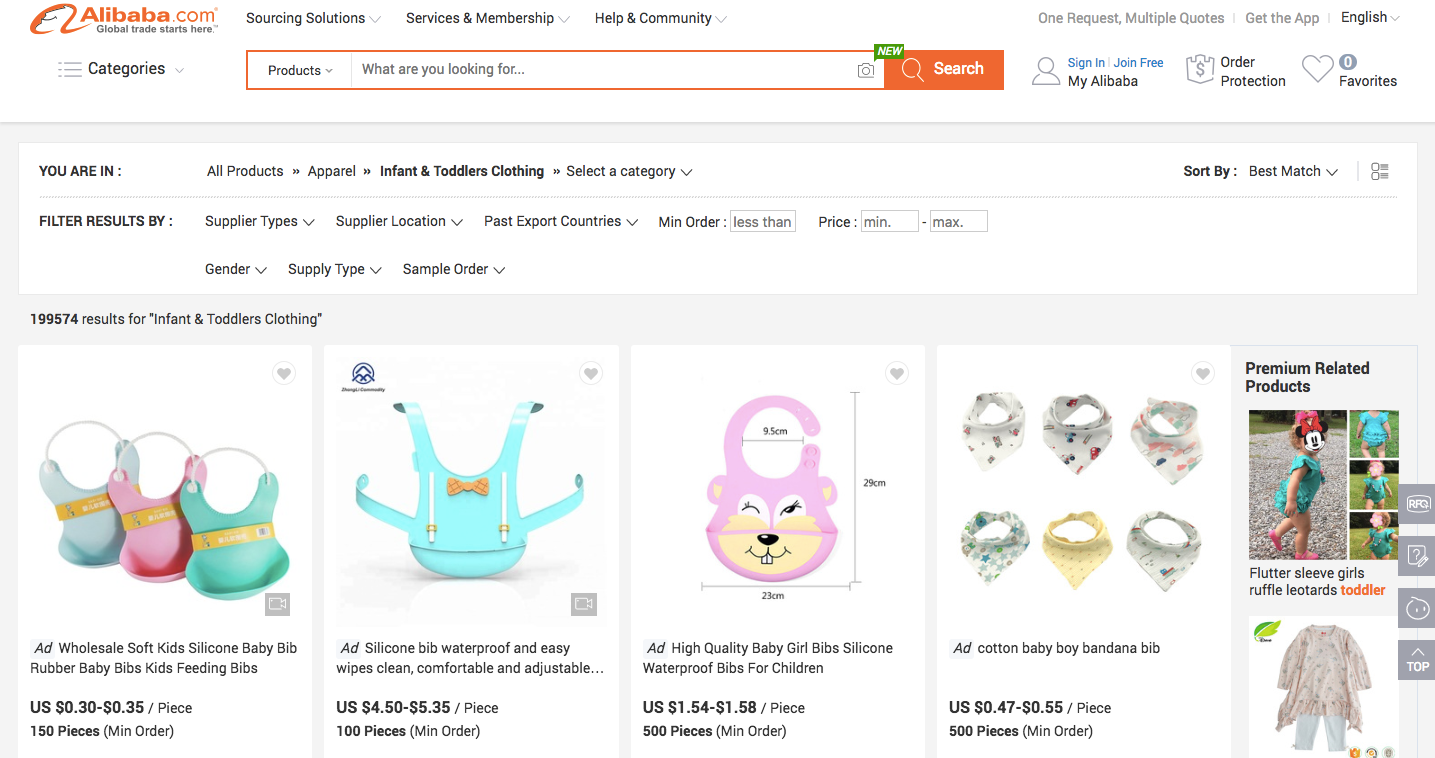The screenshot from Alibaba.com prominently features a webpage geared towards global trade. Displayed in the top left corner is the Alibaba logo in orange, accompanied by the tagline "Global Trade Starts Here." To the right of the logo, the navigation bar lists options such as "Sourcing Solutions," "Services & Membership," and "Helping Community." Further right, a prompt reads "One request, multiple quotes," with additional prompts to "Get the App" and a language selector set to English.

Below this navigation bar, an orange section highlights a search bar labeled "What are you looking for?" with an adjacent "Search" button in orange. To the right, user account options are available, including "Sign In," "Join Free," "My Alibaba," "Order Protection," and "Favorites."

The main content area is dedicated to product listings, starting with the breadcrumb navigation indicating the user is viewing "All Products > Apparel > Infant & Toddler Clothing." Various filters are available on the left side, allowing for refinement by supplier type, location, past export countries, minimum order, price, gender, supply type, and sample orders. 

The results section displays a vast number, specifically 1,999,574 listings for infant and toddler clothing. The first five products featured are:
1. A wholesale soft silicone baby bib.
2. Another silicon baby bib in blue.
3. A bib featuring a character that resembles a purple beaver.
4. Colorful, patterned bibs.
5. Bandana-style bibs.

To the right of the product images, additional pictures of related items are shown, emphasizing the diversity of infant and toddler clothing available on the platform.